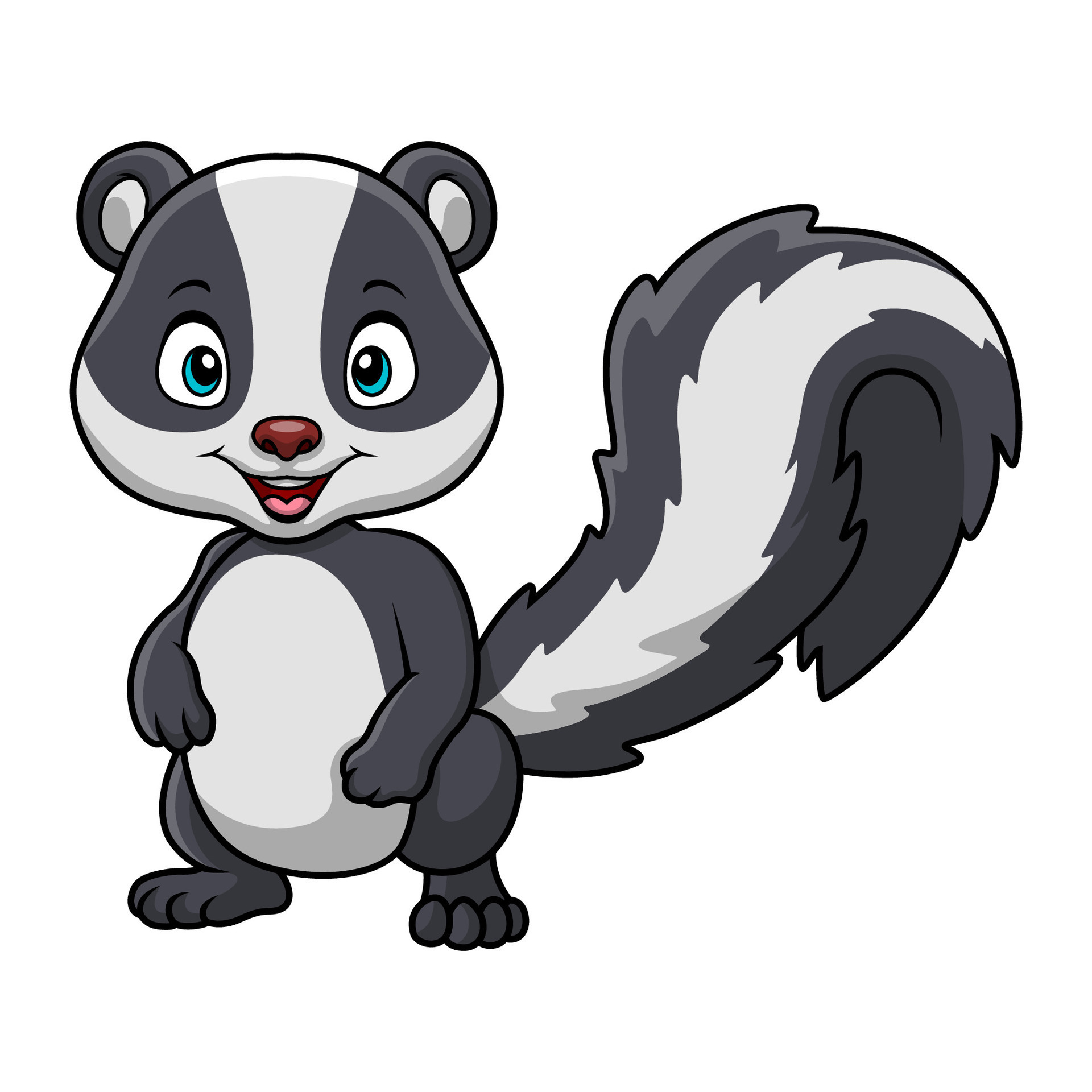The image is of a cartoon skunk, drawn in a quintessential American cartoon style, standing on two legs and looking directly at the camera with a cheerful expression. The skunk features big, expressive turquoise eyes, a brown nose, and red lips, all contributing to its happy demeanor with an open-mouthed smile. The creature has a black and white fur pattern, accentuated by a large white belly and finger-like appendages at the ends of its little black arms and legs. A prominent feature is its long, bushy tail, which has a jagged design with a white stripe running down its center. The background is completely blank, drawing all attention to the charming skunk whose toes on one foot are pointed towards the camera, resembling little egg shapes.